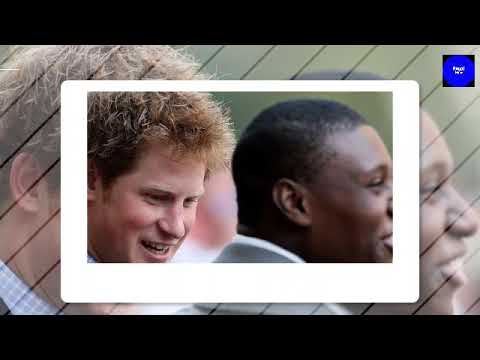This detailed photograph captures a striking composition featuring two men, both framed within a white border, creating a Polaroid-like effect. On the left side of the image, there is a Caucasian male who bears a resemblance to Prince Harry, characterized by his long, slightly spiky red hair, and a smile as he looks downward. On the right side, an African American male with short black hair is also smiling, though his face is partially cut off on the edge of the frame. He appears dressed in a white shirt paired with a gray suit jacket. Behind this foreground image, a larger, slightly blurred version of the same scene serves as a backdrop, with white dashed lines running diagonally across it. The entire image is bracketed by black widescreen bars on the top and bottom, further emphasizing the formal, possibly event-related setting captured outdoors. The dominant colors include shades of brown, pink, tan, white, black, gray, and green.